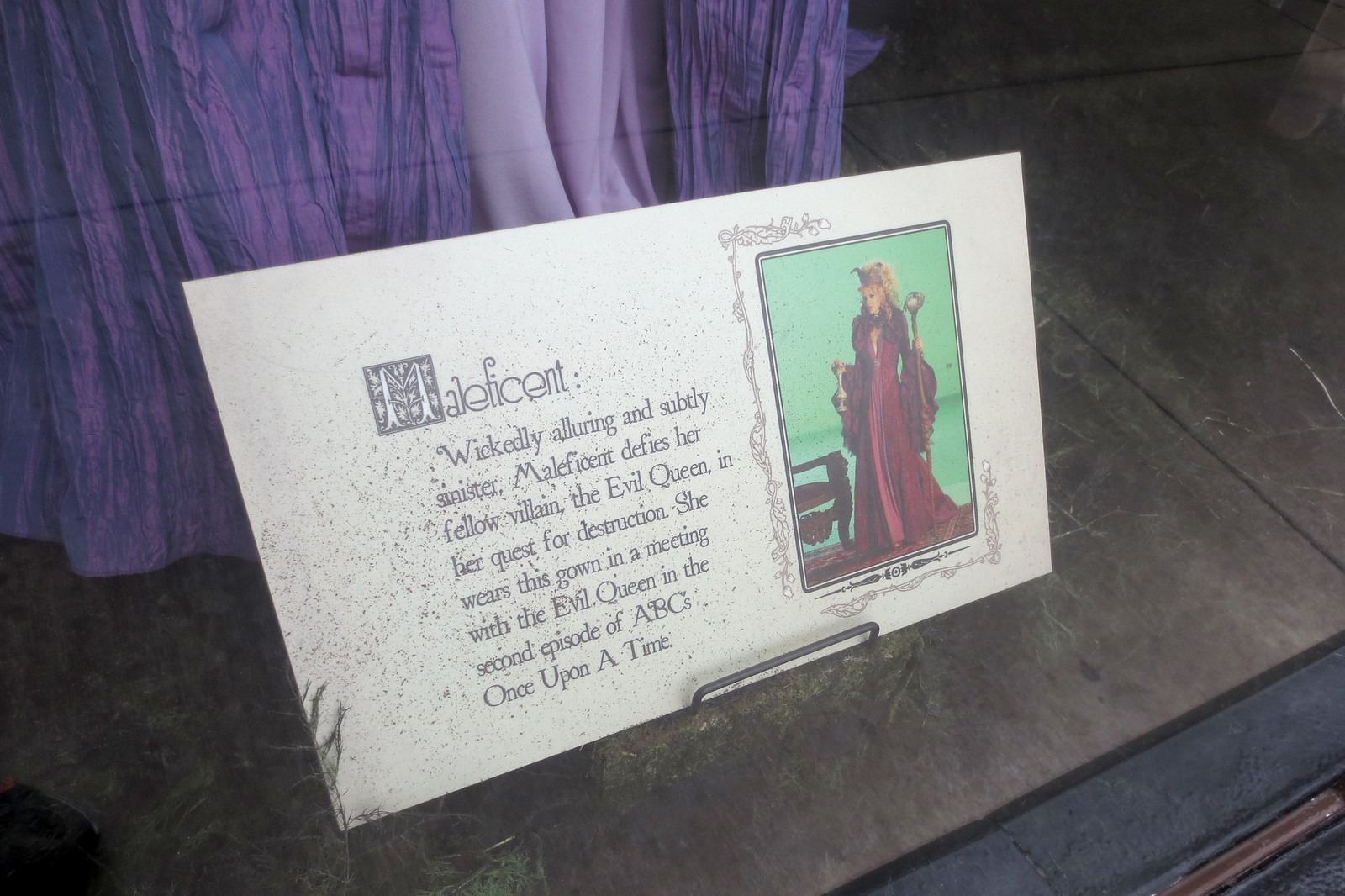This is a detailed photograph of a white placard balanced on a gray, stone-like surface with a purple curtain hanging in the background. The placard, approximately 5 by 10 inches, features black text on the left side that reads: "Maleficent, wickedly alluring and subtly sinister. Maleficent defied her fellow villain, the Evil Queen, in her quest for destruction. She wears this gown in a meeting with the Evil Queen in the second episode of ABC's Once Upon a Time." The text is speckled with black spots which make it slightly difficult to read. On the right side of the placard, set against a green background, is an illustration of a blonde woman dressed in a long purple gown with long sleeves. She is depicted holding a rod or magic wand in her left hand and a bell or container in her right hand. A brown chair is seen next to her. This evocative and detailed scene captures the essence of the character Maleficent from the popular television series.